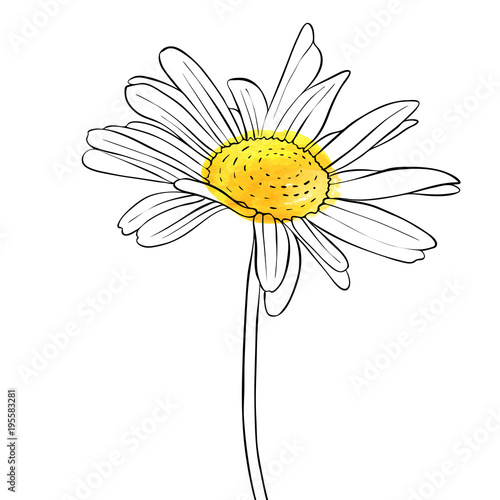The image is a simple yet detailed black-and-white drawing of a daisy, rendered primarily with pencil or pen. The daisy has about 20 long, white petals radiating in different directions from a central yellow core, which appears to be colored with watercolor. The yellow in the center isn't perfectly contained and bleeds slightly onto the petals. The flower creates a subtle 3D effect, adding depth to its form. Despite the minimalistic style, the image includes an Adobe Stock watermark and text on the left side. The overall composition is set against a white background, emphasizing the delicate contrasts in the drawing.